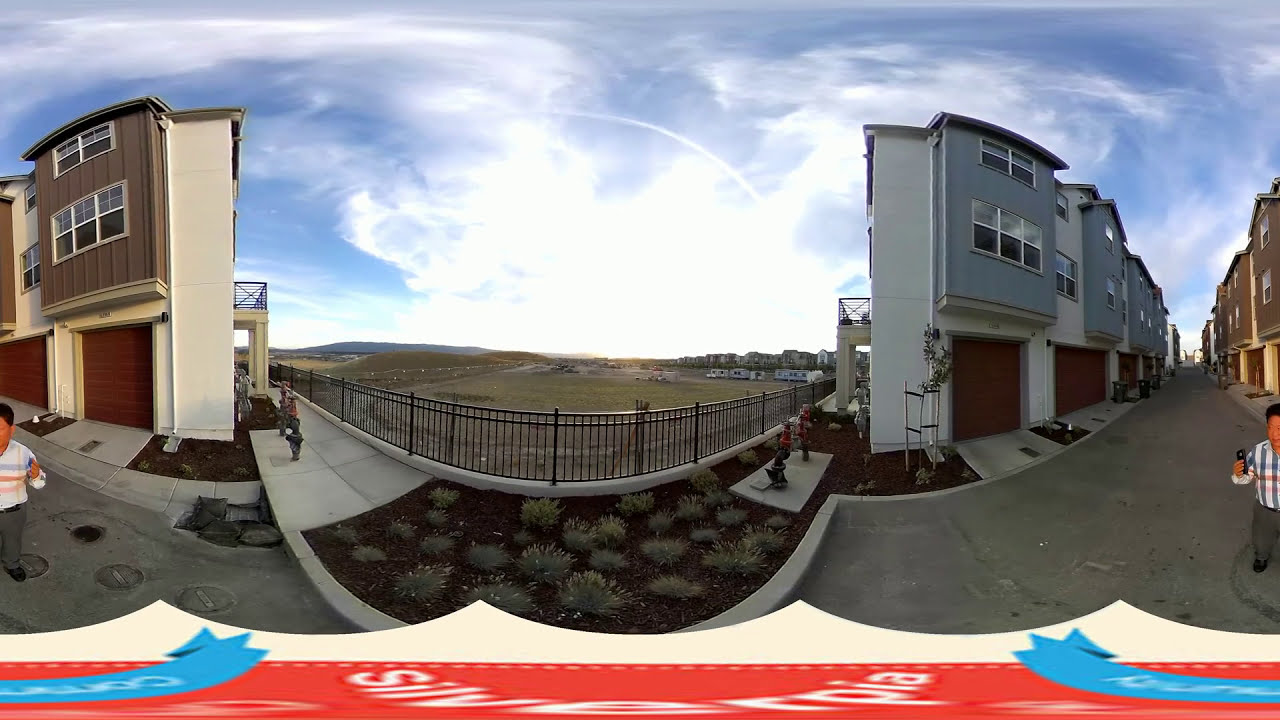The image is a panoramic photograph capturing a charming neighborhood scene centered around an open grassy field with no trees, framed by a black fence and a newly paved white sidewalk. In the midground, one can observe the field's sparse short grass, with distant mountains and a bright blue sky with a few wispy white clouds painting a serene backdrop. On the left, there are brown and tan duplexes with distinct red garage doors; some units feature balconies and small planted bushes enhancing their frontage. On the right side, the row of mostly blue and brown buildings also flaunts red garage doors and similarly small balcony extensions. The duplexes are positioned at a slight angle relative to the street that divides the two sets of townhomes. A man, dressed in a plaid shirt and gray pants, stands at the far right of the photo, holding a cell phone, partly cut off from view. This vivid street view is bordered at the bottom by a red stripe and blue banners, adding a touch of structure to the scene.